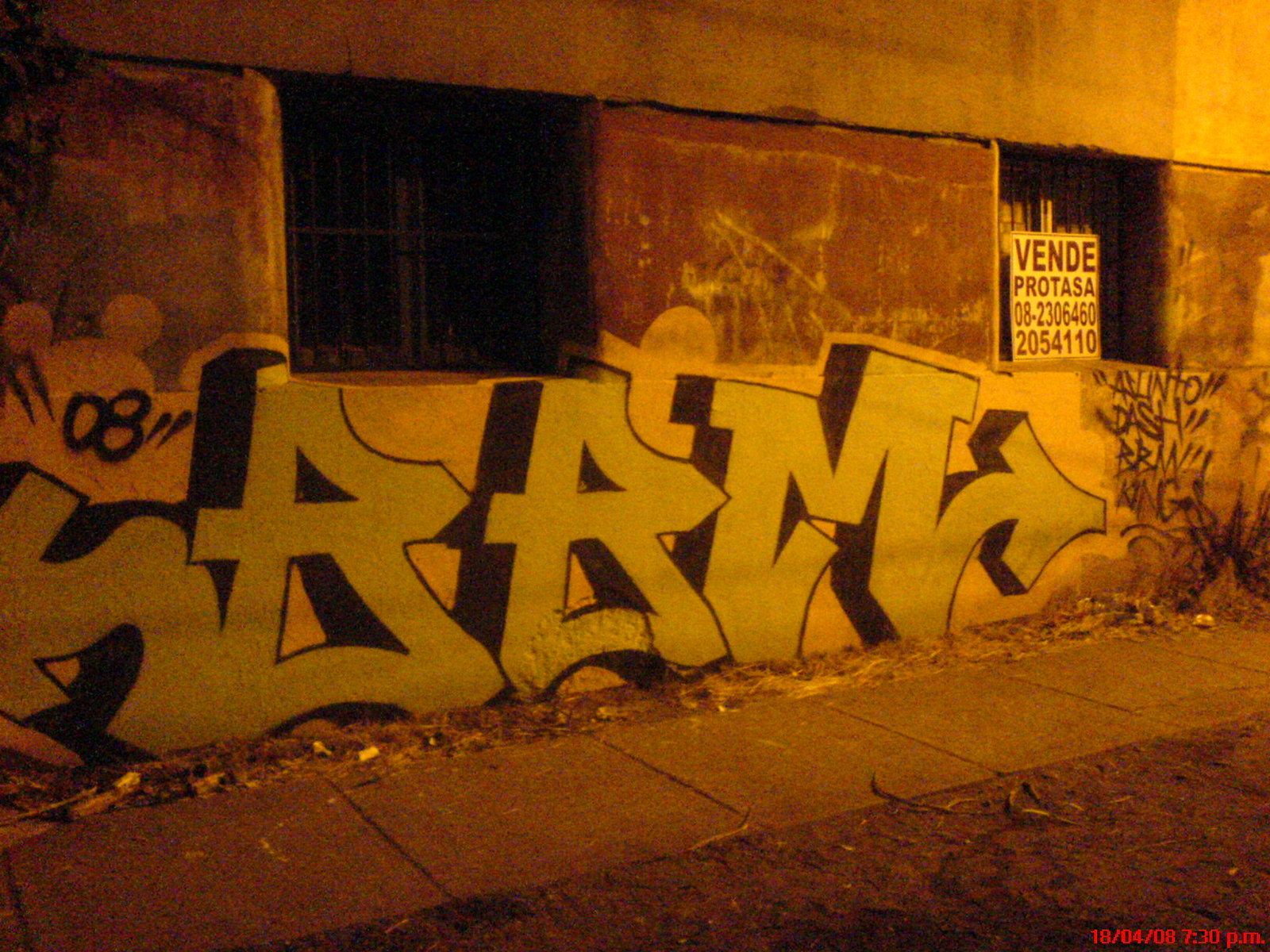This image captures a scene at night featuring a side of a concrete building adorned with graffiti. The structure has two barred windows, with one window on the right displaying a sign in Spanish that reads "Vendee Protassa" followed by phone numbers "08-2306-460" and "205-4110." The graffiti itself is composed of large, 3D stylized letters, predominantly black and light blue against a white background, spelling out "SARM" with arrows integrated into the design. Additionally, "08-08" is written above the tagged letters in quotation marks. A concrete sidewalk runs in front of the wall, and the ground is littered with small bits of trash. The scene is illuminated by a yellow light, giving the entire image a distinct nighttime atmosphere. In the bottom right corner of the wall, the text "1804-08-730 PM" is written in red. The overall setting suggests this is in a non-English speaking country.